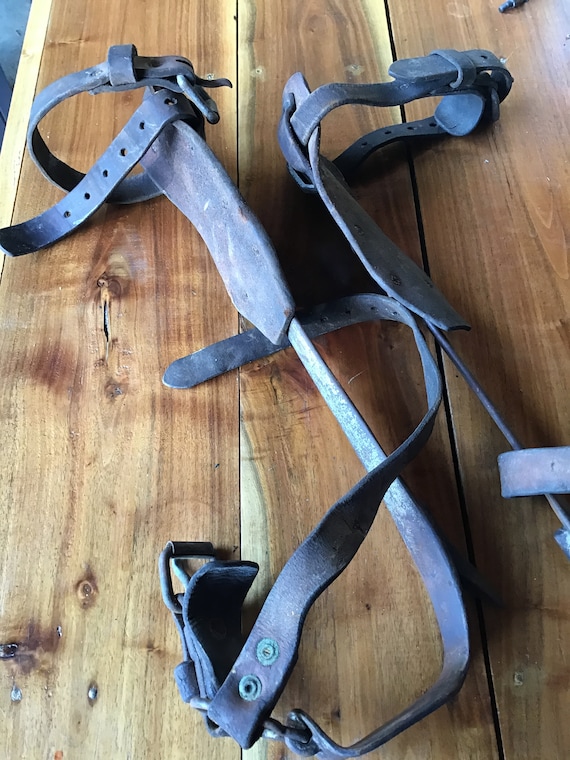This image depicts a pair of worn, equestrian stirrups or foot straps, which are lying on a rustic wooden table composed of three distinct planks. The wood has a medium brown tone with white streaks, showing signs of wear and dings. The straps are predominantly made of black or very dark brown leather that appears dirty and faded with use. Each stirrup features a long, curved metal shaft that forms an L-shape to support the foot. Attached are several leather straps, including one with multiple holes for adjustment and another with a belted cuff at the top, providing extra padding around the leg. The buckles on these straps are fastened and show signs of wear. One stirrup lies facing to the left, while the other is positioned identically but facing the opposite direction.